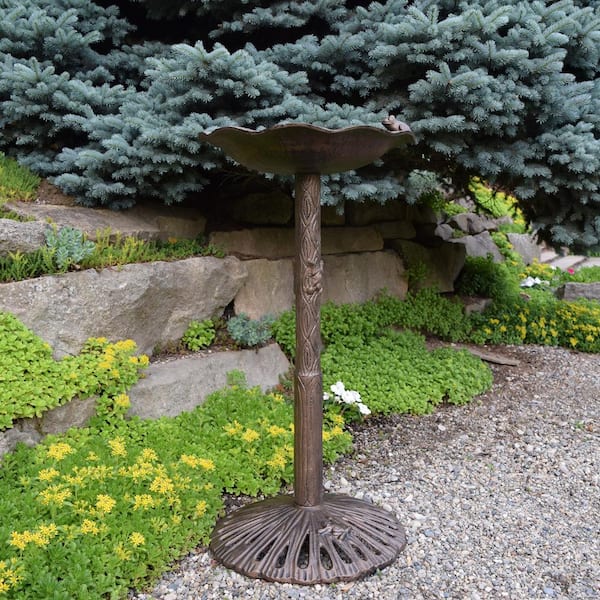This color photograph captures a serene garden scene centered around an ornate birdbath. The birdbath, crafted from a bronze-colored metal, stands tall with a circular, intricately engraved base and a decorative two-part stem. Its bowl-shaped top features a wavy, ruffled edge, and perched gracefully on this rim is a small sculpture of a frog. The birdbath is set upon a foundation of gray gravel, surrounded by various garden elements. In the background, the dense green foliage of a pine tree, possibly a blue spruce, stretches upward, its bristly needles creating a lush canopy. Below the tree, large, square granite rocks form a stone wall, interspersed with petite, light green plants dotted with tiny white flowers. The entire scene is bathed in shades of green, making the birdbath blend seamlessly into its natural surroundings.